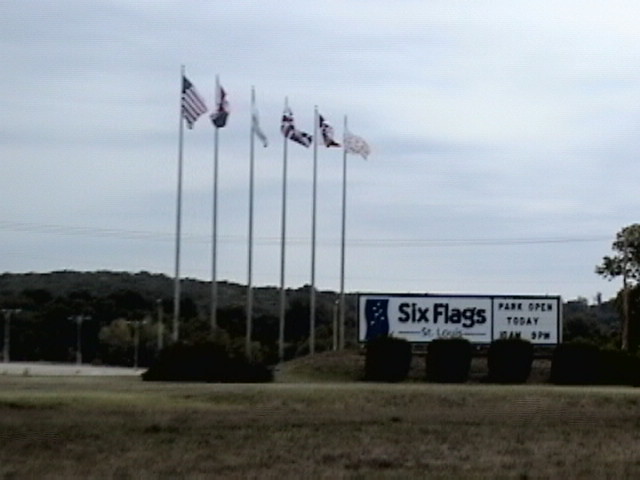In this color photograph taken on an overcast day, we see the entrance gate to Six Flags St. Louis. Dominating the image are six tall flagpoles, each bearing a flag. The flag on the far left is identifiable as the United States flag, with stars and stripes, while the flag in the middle resembles that of Great Britain. The other flags are indiscernible due to the wind blowing them in various directions. Below the flags, there is a sizable rectangular sign reading "Six Flags St. Louis" in black lettering, with additional text indicating "Park open today 10 a.m. to 9 p.m." In the foreground, patches of light brown grass and lush green bushes are visible, though their details are obscured by shadows. A green, tree-covered hill is faintly visible in the background, along with a pale road cutting through the landscape. The sky overhead is light gray, contributing to the overall dark and blurry quality of the image, which might suggest it was taken with an older digital camera.